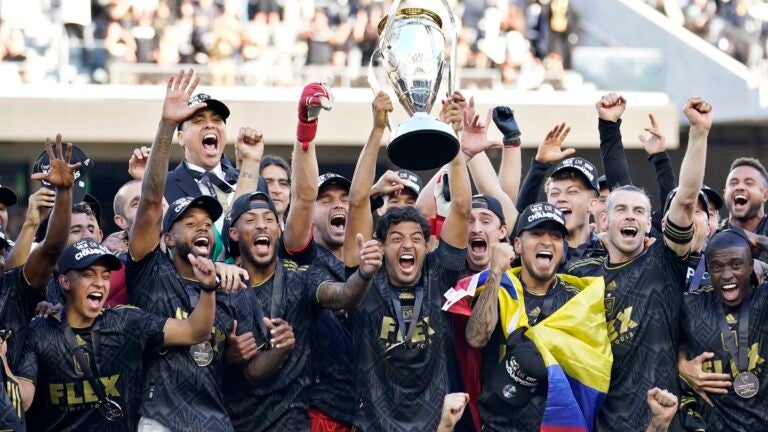In the center of the photo, a group of jubilant athletes, likely from a soccer or sports team, are celebrating their victory on a field. The team members are all clustered together, shoulder to shoulder, with most of them lifting their right hands triumphantly into the air. They are all wearing black jerseys adorned with medals, each hanging from a black strap, indicating their recent achievement. The central figure, a dark-skinned man, holds a large, silver, cone-shaped trophy above his head, his mouth wide open in a scream of victory. To his right, a man draped in yellow, blue, and red striped flag stands proudly, also holding up his hand. The background reveals a few blurry bleachers with spectators and a beige wall. The image captures the exuberance and diversity of the team in their moment of triumph.